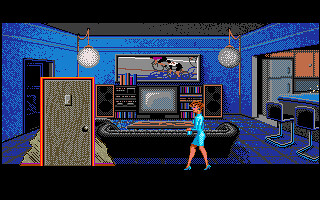This image appears to be a screenshot from a pixel art style computer game, likely designed to evoke the aesthetics of the 80s or 90s. The scene displays a room rendered in detailed, colorful pixels, showcasing a blend of modern and retro elements. Dominated by blue hues, the room features a gray ceiling and includes distinctive orange metal posts with chandelier-style lights hanging from them. The central focus is a woman with short red hair—though some descriptions note it as brown—dressed in a blue dress and matching blue heels, walking to the left.

In the background, a television is flanked by large black stereo speakers accented with orange and additional stereo equipment. Beneath a rectangular picture frame on the wall, there's a sound system. The room's gray door, bordered in contrasting red, stands out on the left side. To the right, a partition reveals an adjacent kitchen area with a gray refrigerator, peach-colored cabinets, and a seating area featuring black metal-framed chairs in front of a blue bar. This image seamlessly blends different room elements, capturing both a nostalgic and contemporary feel, indicative of a carefully designed gaming environment.